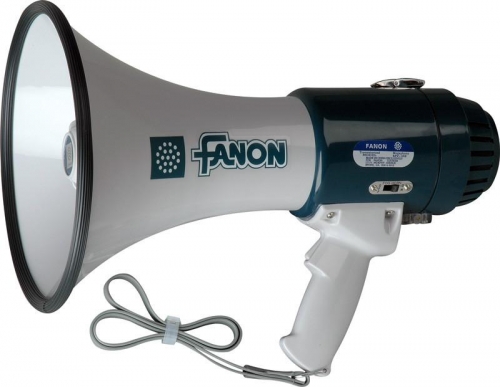The image depicts a handheld megaphone labeled with the brand name FANON. The megaphone is positioned on its side, directing its large circular horn opening towards the left, which is bordered in black with a white interior. As the horn narrows into a cylindrical shape, the FANON brand name and logo are visibly printed on this section. The primary structure of the megaphone is predominantly white except for the area from which the words are spoken, which is dark blue or green. Below the main body, there is a white handle and a gray cord extending from it. Additionally, a metal plate with a plastic on-off switch is located above the handle. The background of the image is plain white, accentuating the details of the megaphone.